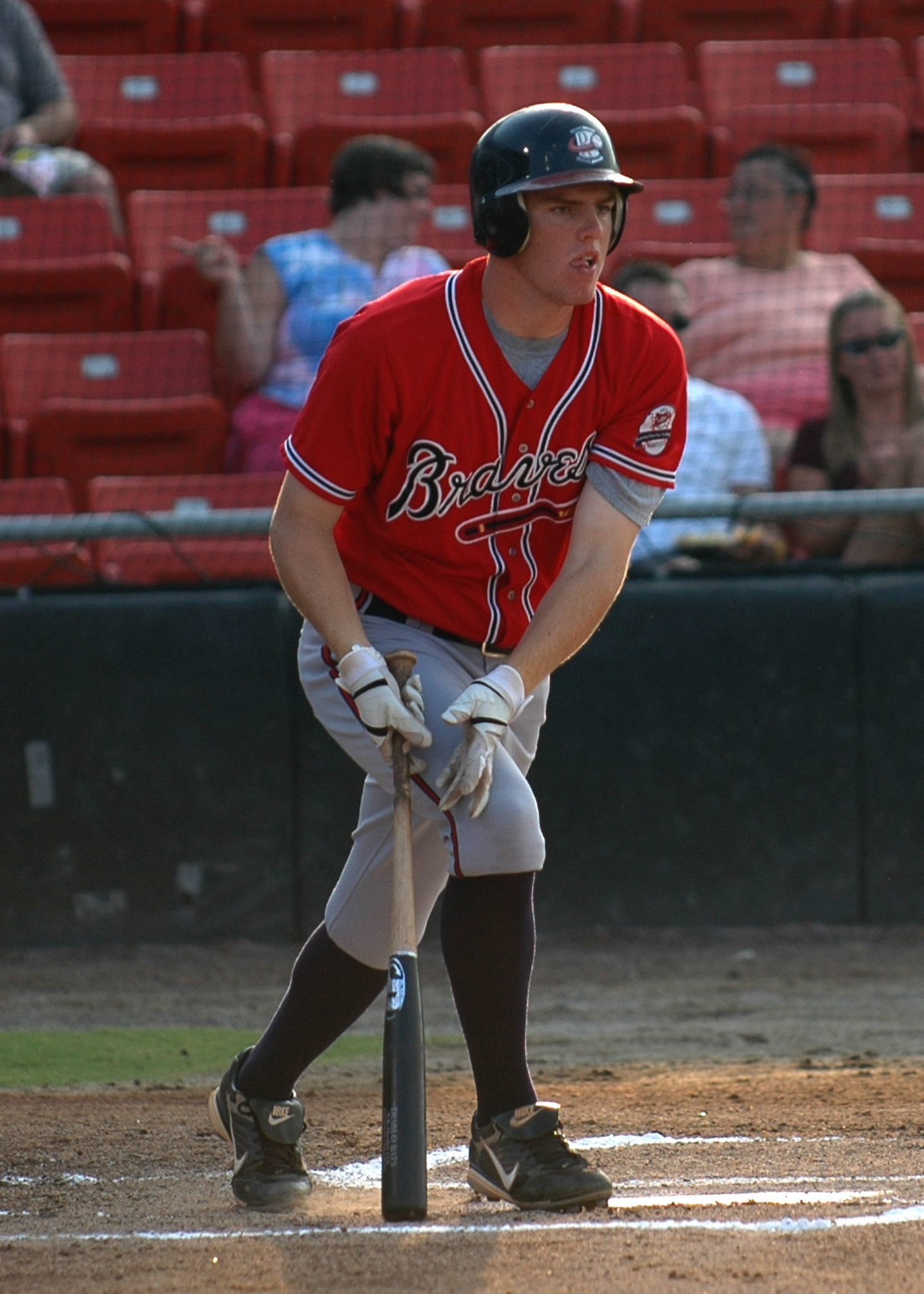This detailed and vibrant outdoor, daylight photograph captures a young white male baseball player standing at home plate. He is adorned in a distinctive athletic outfit, including a black batting helmet, a red button-up jersey with "Braves" written across it, gray pants, black socks, and black athletic shoes. His hands are protected by white batting gloves as he grips a bat with a black top and a brown handle, poised to either take a swing or setting up for one, with the bat resting at his side. The player is surrounded by a cloud of dust, highlighting his readiness and action.

Situated at home plate within the batter's box, the scene is framed by a short padded brown wall and a protective black net. Behind this setup, several women can be seen sitting in rows of red bleachers, which feature gray name tags in the middle of their backs. Among them are two older women and a younger woman in the front row, along with another partially obscured person. The detailed scene captures the essence of a lively baseball game, with the player's focus and the spectators' engagement enhancing the overall atmosphere.